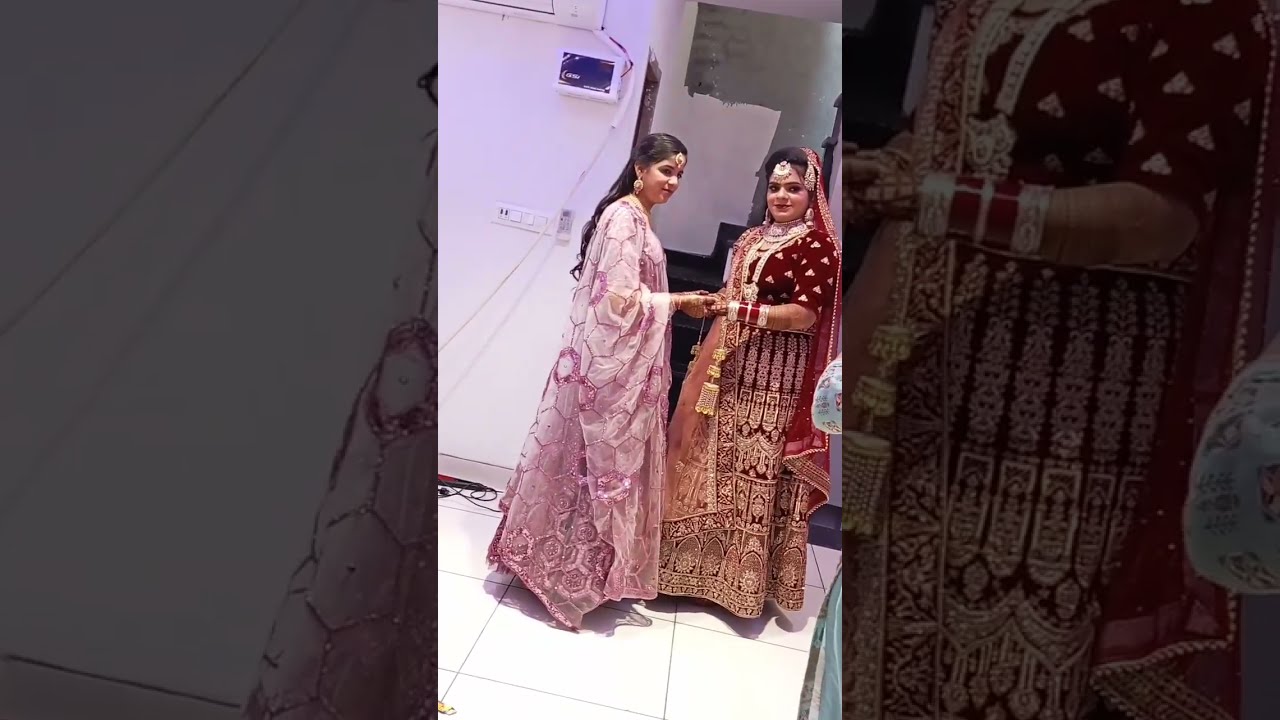This horizontally rectangular image features two Indian women standing and facing each other while holding hands, though both are looking toward the camera and smiling. They are dressed in elaborate traditional gowns. The woman on the left is wearing a long, pink gown with geometric prints; she has long black hair that cascades down to her waist and is adorned with a gold forehead piece and large dangly earrings. The woman on the right is dressed in a red and gold gown and wears a similar gold forehead piece and long dangly earrings. She also has numerous red bracelets on her wrist and a red veil. The sections on the left and right of the image are grayed out, featuring close-ups of the pink gown on the left and the red and gold gown on the right. In the background, there is a wall with some wiring and boxes, and they are standing on a white tile floor. Partially visible on the right is another person in a bluish-colored dress, cut off by the frame. The overall scene hints at a celebratory or ceremonial occasion, possibly a wedding.